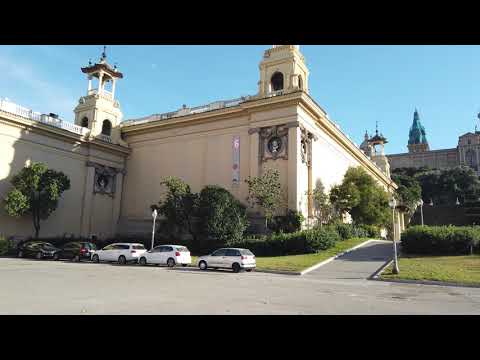The image depicts an outdoor setting framed by thick black borders at the top and bottom. Dominating the scene is a grand, rectangular building that appears to be a cathedral or church. This imposing structure, located towards the left-center of the image, boasts tall, light sandstone walls adorned with intricate details. The building features numerous spires, including small towers with rounded openings at their tops. In the foreground, in front of the building, a gray asphalt road or driveway stretches across the scene, with two dark-colored cars and three white-colored cars parked on it.

To the right side of the primary building, a path lined with trees and bushes leads towards another taller structure in the background. This second building, identifiable by its distinctive blue, pointed spire, rises above the surrounding trees. The sky above is a bright blue, dotted with patches of white clouds, adding to the overall tranquility of the scene.